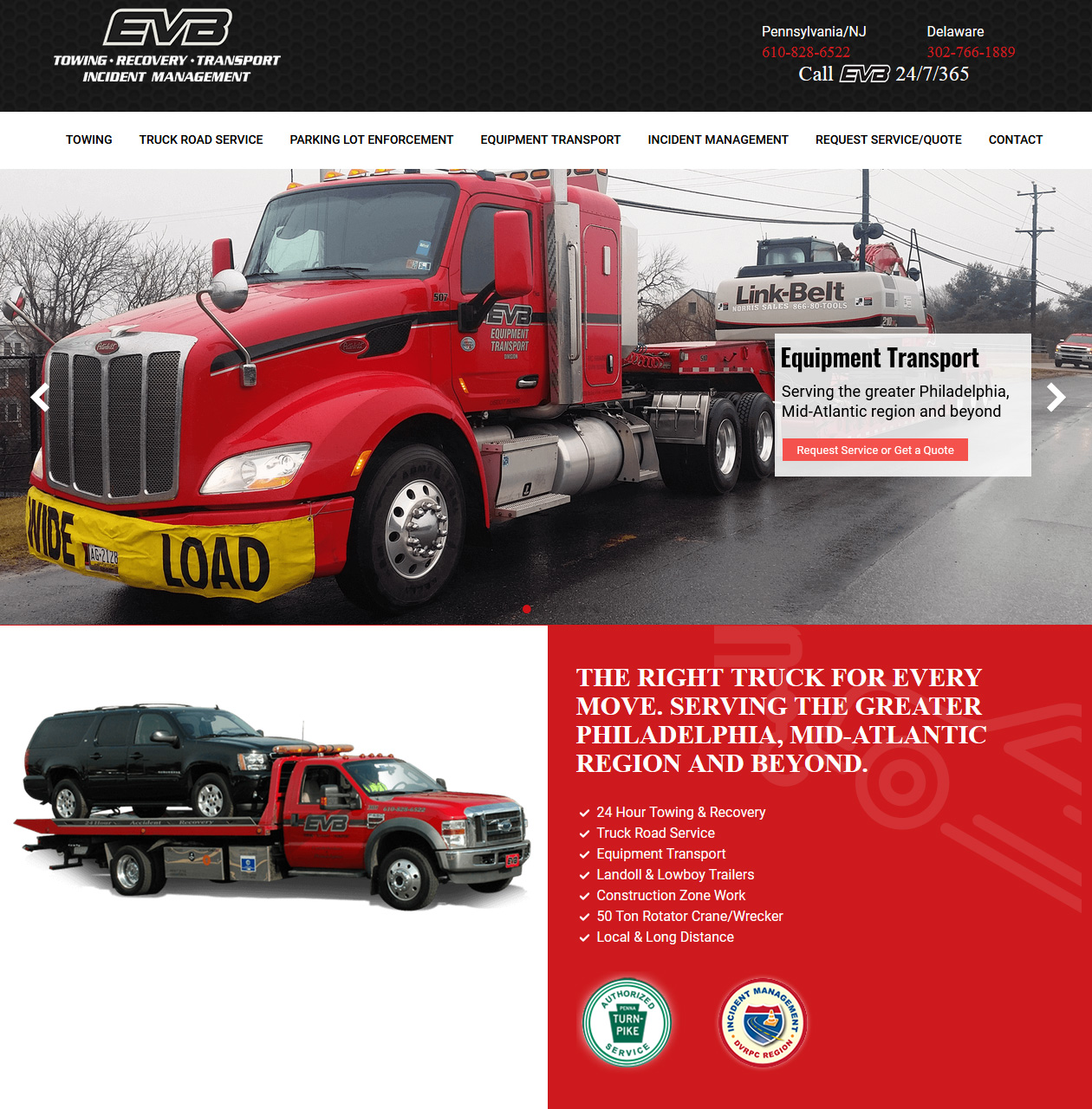The image is a detailed website for a trucking company. At the top of the webpage, a black border spans the header, with "EVB" prominently displayed in the upper left-hand corner. Beneath that, the text reads "Towing, Recovery, Transport, Incident Management." To the right, it lists the service areas: Pennsylvania, New Jersey, and Delaware, along with a call-to-action: "Call EVB 24-7-365."

Directly below is a menu bar with the following options: Towing, Truck Road Service, Parking Lot Enforcement, Equipment Transport, Incident Management, Request Service/Quote, and Contact. The main visual feature of the page is a large, horizontally-stretching image of a red semi-truck adorned with a yellow "WIDE LOAD" banner across its bumper, transporting heavy equipment on a road. In the bottom right corner of this image, a white square reads "Equipment Transport."

At the lower left corner of the screen, there's another white box displaying an image of a red truck pulling a red trailer, which is transporting a black SUV on its flatbed. Next to this, another white box contains the text: "The Right Truck for Every Move, Serving the Greater Philadelphia, Mid-Atlantic Region and Beyond, 24-Hour Towing and Recovery, Truck Road Service, Equipment Transport, Landoll and Low Boy Trailers, Construction Zone Work, 50-Ton Rotator Crane Wrecker, Local and Long Distance."

Two circular badges appear towards the right; one reads "Authorized Service," while the other seems to say "Incident Management, Certification Required."